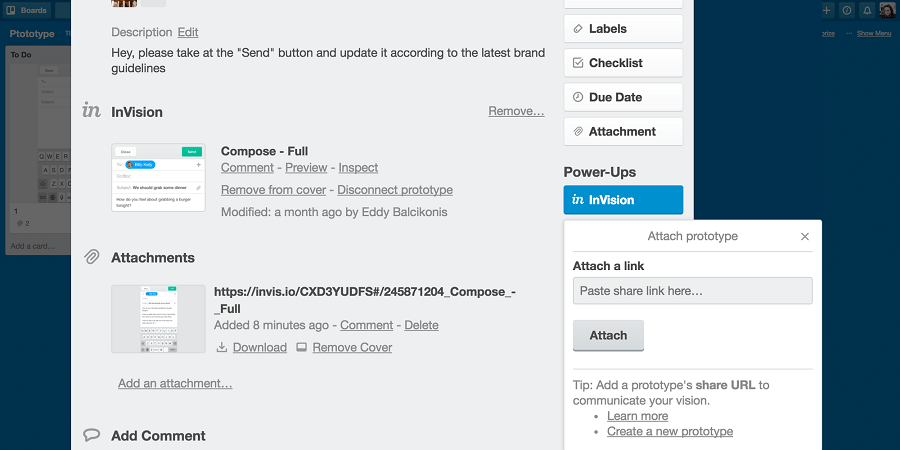An image of a website page displays a detailed description with various interactive elements and attachments. At the top of the page, there is a message reading, "Hey, please take at the send button and update it according to the latest brand guidelines," suggesting a possible typo, with "take at" likely intended to be "take out." Below this message, several buttons are visible bearing the labels: "Envision," "Compose," "Full," "Comment," "Preview," "Inspect," "Remove from Cover," and "Disconnect Prototype."

The page indicates that the content was modified a month ago by Eddie Bell-Sinokas. Furthermore, an "Attachments" section features a prominent attachment link, accompanied by a thumbnail image. The text highlights that the attachment was added eight minutes ago. Underneath, an option to "Add an Attachment" is visible.

On the right side of the page, there is a pop-up box labeled "Attach Prototype." Within this box are fields for "Add a Link" and "Paste Share Link Here," along with an "Attach" button for finalizing the attachment process. The well-organized layout provides clear information regarding specific actions, contributions, and recent updates.